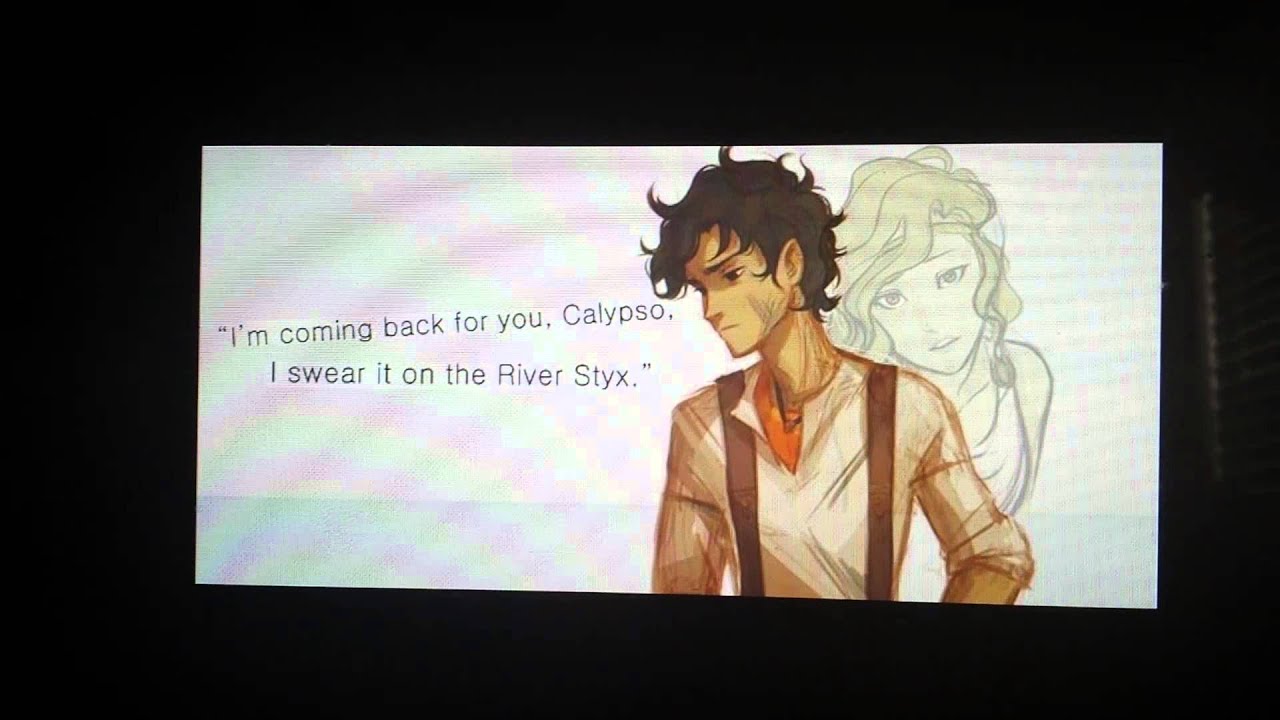The image is a detailed piece of art featuring two characters and some text. On the left side of the image, a poignant quote reads: "I'm coming back for you, Calypso. I swear it on the river Styx." 

To the right of the text, the main focus of the artwork is a boy who appears to be in his teenage years. He has a rugged appearance with dirt marks on his face, suggesting he's been through a lot or possibly works a labor-intensive job, perhaps as a farmer. His brown hair is messy, either from natural curls or from being tousled. The boy's expression is filled with worry or disappointment, as he gazes downward and to the left. His attire includes a simple white shirt and black trousers, secured with black suspender straps over his shoulders.

Standing directly behind the boy is a blonde girl, who is likely Calypso, given the context of the quote. Her expression mirrors his, laden with concern as she looks at him intently from behind. The close proximity and her worried gaze suggest a deep connection between the two characters, likely influenced by the boy's vow in the quote.